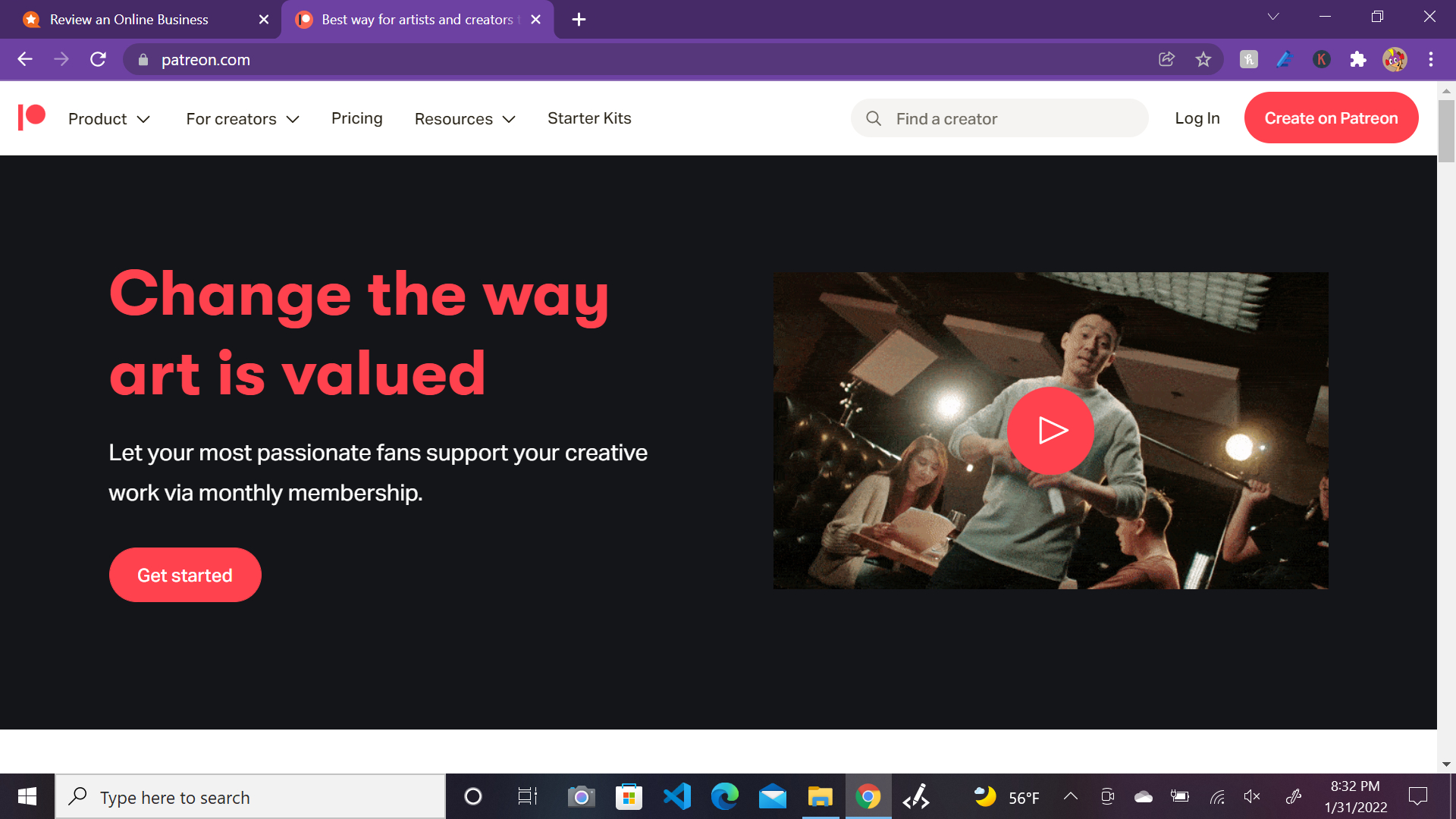This image depicts a webpage with several distinct elements. At the very top of the page, there is a navigation menu featuring multiple items. The text appears quite small and difficult to read, but the highlighted item is in purple and seems to include the phrase "best way for artists." The menu also contains an entry mentioning "patreon.com," though this is also challenging to decipher.

Below the navigation bar, there is a white area with various interactive elements from left to right. On the far left, there is a red icon consisting of a vertical red line next to a circle. Following this, there are several menu items: "Product" with a dropdown icon, "For Creators" with a dropdown icon, "Pricing," "Resources" with a dropdown icon, and "Starter Kits." Next to these, there is a search box with a magnifying glass icon and the placeholder text "Find a creator." This is followed by a "Login" option and a red oval button with white lettering that reads "Create on Patreon."

The remainder of the page has a black background. On the left side, there is a bold message in bright red font that reads "Change the way art is valued." Below this message, white text invites users to "Let your most passionate fans support your creative work via monthly membership." Directly beneath this invitation, there's a red oval button with white lettering that says, "Get Started."

On the right side of the page, there is a prominent horizontal rectangular video thumbnail. The thumbnail features a play button in the center, indicating that it is a video. In the video, a man is centered with a circle play button on him. In the background, there are additional people, including a woman and another individual. A camera is visibly focused on the man.

Below the video thumbnail, there is a bar that includes a white search box with a magnifying glass icon on the left side and black placeholder text. This bar also contains several small computer icons.

In summary, this webpage appears to be offering artists a platform for receiving support from their fans via monthly memberships, likely through Patreon, with various interactive elements and a promotional video to elaborate on the service.